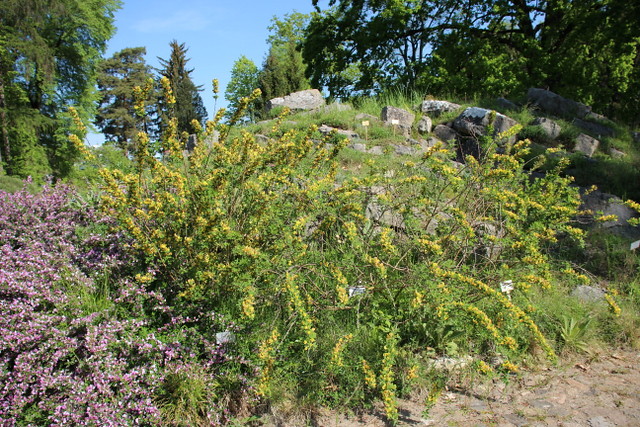In the foreground of this daytime photo, a vibrant garden area is showcased. Dominating the scene are two prominent bushes amidst a sandy and rocky ground. On the left, a compact bush boasts tightly clustered, small purple flowers interspersed with hints of white and green stalks peeking through. In contrast, the bush on the right is more free-form, with long green stalks adorned with tightly bound clusters of bright yellow flowers. Tall grass is visible, growing around and through both bushes, particularly noticeable amidst the purple flowers.

In the middle ground, a patch of light brown dirt separates the bushes from a small rocky hillside. The hillside, located in the back right corner, ascends gently with rocks dispersed throughout. Little signposts with white labels are placed at the base of both the yellow and purple bushes, with a couple more signs spotted on the hillside.

Surrounding the entire area is a dense tree line of large trees, framed against a bright blue sky devoid of clouds. Sun rays cast subtle shadows on parts of the ground, enhancing the scene's natural and serene ambiance.